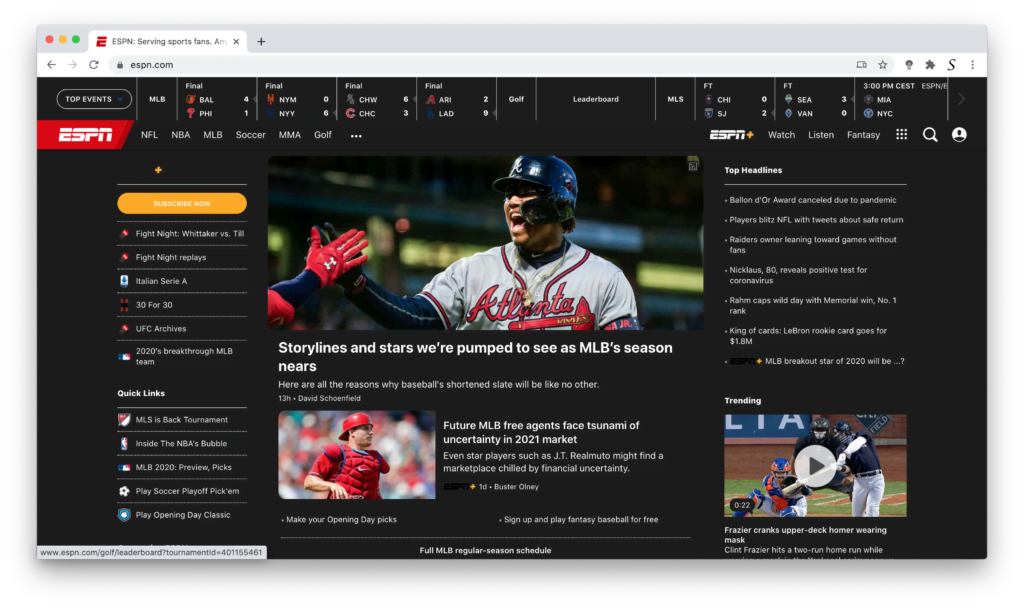This image captures the homepage of ESPN's website. The topmost border is a sleek gray strip about half an inch thick. On the left side of this border, there are three colored dots: a red dot, a yellow dot, and a green dot, reminiscent of standard window control buttons. Adjacent to these dots is a protruding white tab extending about two inches inward. Within this white tab, there is a bold red letter "E," followed by the black text "ESPN, serving sports fans." The trailing period is immediately followed by the letter "A" before the text abruptly ends. Adjacent to this, there is a black "X" icon for closure, and right next to it, a black "+" sign.

Beneath the gray border, a white navigation strip features an arrow pointing left, an arrow pointing right, a refresh icon, and a search bar. Inside the search bar sits a small lock icon followed by the text "ESPN.com." To the right of this search bar are star and share buttons. 

The main body of the webpage is predominantly black. At the very top, a black tab bordered in white bears the label "Top Events," listing scores from various games. At the center, there's a "Leaderboard" indicator. Below this, there's a prominent red tab inscribed with "ESPN" in white, flanked by the names of different sports in white lettering: NFL, NBA, MLB, Soccer, MMA, Golf, and an icon with three ellipses indicating more options.

Along the left side, there is a column providing quick links and a "Subscribe Now" button, interspersed with information about upcoming events like "30 for 30." Below this column, there's an image featuring an 11th Braves player. Beneath this image, the text reads "Storylines and Stars We’re Pumped to See as MLB Season Nears," presented in white. Following this heading, there are two lines of text next to an image of a catcher dressed entirely in red, accompanied by about four lines of white text providing further details.

On the right side of the page, the section titled "Top Headlines" is clearly marked in white. Below a thin grey divider, there are seven listed headlines. In the bottom right corner of the page, a video thumbnail shows a player swinging a baseball bat, alongside three lines of descriptive text in white.